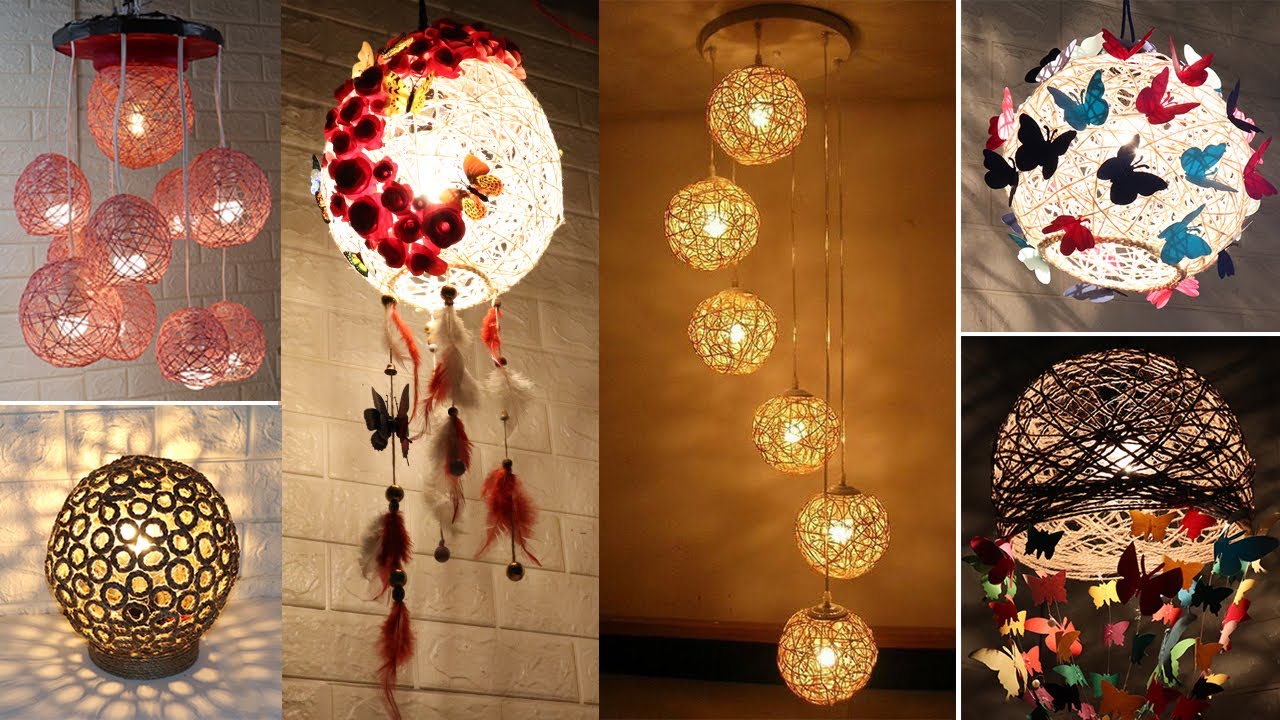The horizontal rectangular image is a collage composed of several smaller rectangular images, each highlighting a variety of decorative light fixtures. In the upper left corner, there is a chandelier-like light with pink globes hanging at various heights, each featuring a central light bulb. Below this, there is a table lamp designed like a globe with intricate patterns. Adjacent to this is a full-length rectangular section depicting a dreamcatcher adorned with numerous feathers. To the right, another hanging light fixture descends from the ceiling, showcasing six golden globes in succession, each encasing a light bulb. Continuing right, there is another section divided into two parts. The upper part shows a lit orb surrounded by colorful butterflies, while the lower part features a wicker basket-shaped light fixture with light bulbs and butterflies emerging from it. The entire collage feels like a catalog page, presenting a variety of aesthetically pleasing lights, some spherical with starched thread patterns, many with an added flourish of butterflies or feathers, each intricately detailed and evocatively displayed.